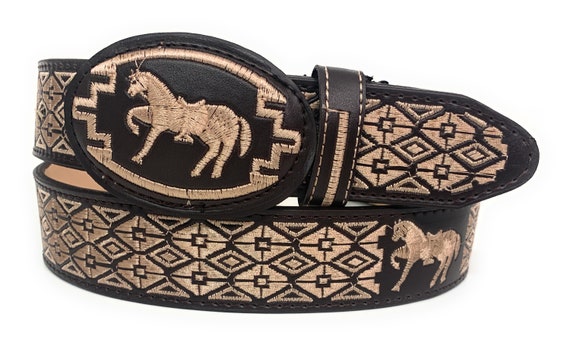The image depicts a rolled-up black leather belt set against a plain white background, showcasing both a top and a bottom loop. The belt features an intricate design embroidered in tan and white thread. A repeated pattern of diamonds and triangles runs uniformly across the belt, each diamond intricately detailed with lines and squares. Central to its design, a prancing horse motif, with one front leg raised and a saddle on its back, appears prominently in two locations: on the bottom loop and framed within an oval pattern on the top loop near the buckle. The belt buckle itself mirrors this motif, featuring the same stitched horse design encircled by a zigzag pattern. The craftsmanship suggests a piece from the late 1800s to early 1900s, possibly from the Western United States, hinting at its use by a cowboy.